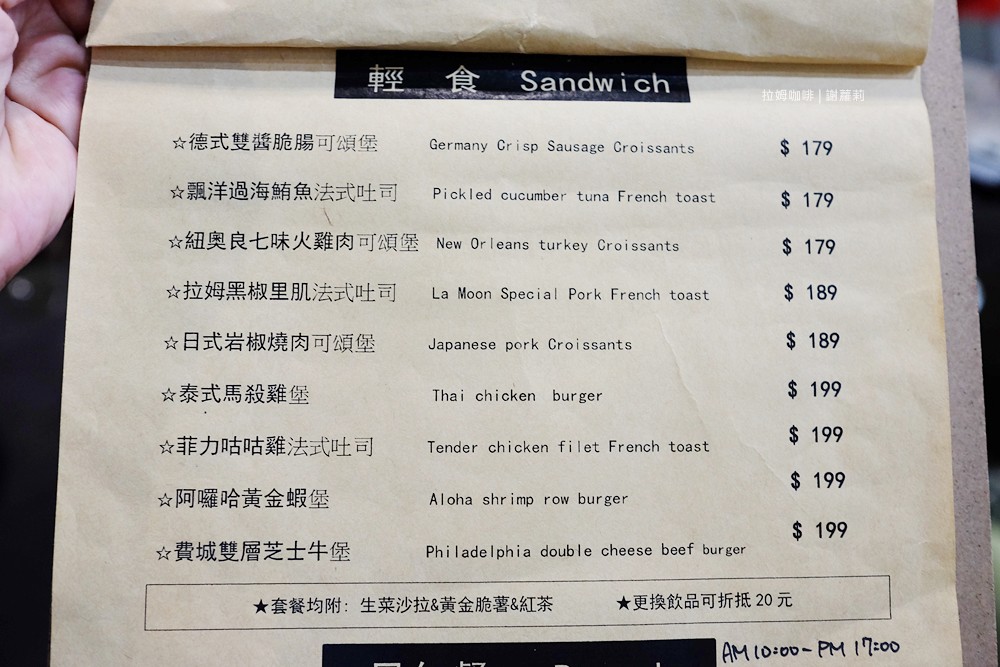The image displays a menu with the word "SANDWICH" prominently printed at the top within a black rectangle. The menu is bilingual, featuring Chinese characters on the left side and their corresponding English translations directly to the right. Prices are listed on the far right. The menu items, from top to bottom, include:

1. Germany Crisp Sausage Croissants - $179
2. Pickled Cucumber Tuna French Toast - $179
3. New Orleans Turkey Croissants - $179
4. Le Moon Special Pork French Toast - $189
5. Japanese Pork Croissants - $189
6. Thai Chicken Burger - $199
7. Tender Chicken Filet French Toast - $199
8. Aloha Shrimp Roe Burger - $199
9. Philadelphia Double Cheese Beef Burger - $199

Next to each menu item's Chinese name, there is an outlined but unfilled star. The hours of operation, handwritten at the bottom right corner, are indicated as 10:00 AM to 5:00 PM, with "5:00 PM" represented as "17:00" in 24-hour format.